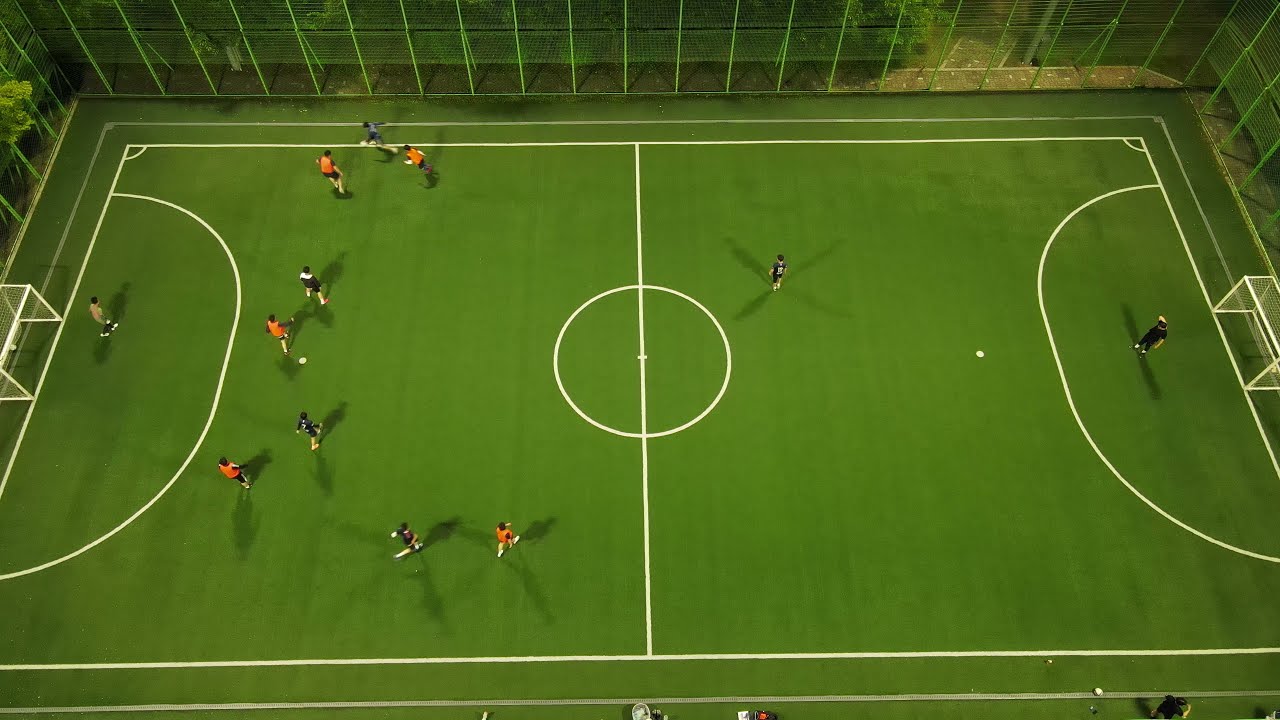This color photograph, taken from an aerial perspective, captures a nighttime soccer match on a small, well-defined green field surrounded by a tall green fence. The field is marked with white lines, featuring goals at each end, a central circle, and defined goal areas. The scene is primarily illuminated from overhead lights, revealing the players and the nearby surroundings. Trees are visible just beyond the fence, adding to the scenic outdoor setting. 

On the left side of the field, a significant cluster of players from both teams—wearing either blue and black or orange and black jerseys—are densely gathered, presumably contesting the ball. The blue team's goalkeeper stands solitary on the right side of the field, while the orange team's goalkeeper is positioned on the left. In total, there are about 10 to 12 players actively engaged in the game.

In the bottom area of the photograph, a few spectators can be seen watching the match from the sidelines, adding a communal touch to the athletic event.